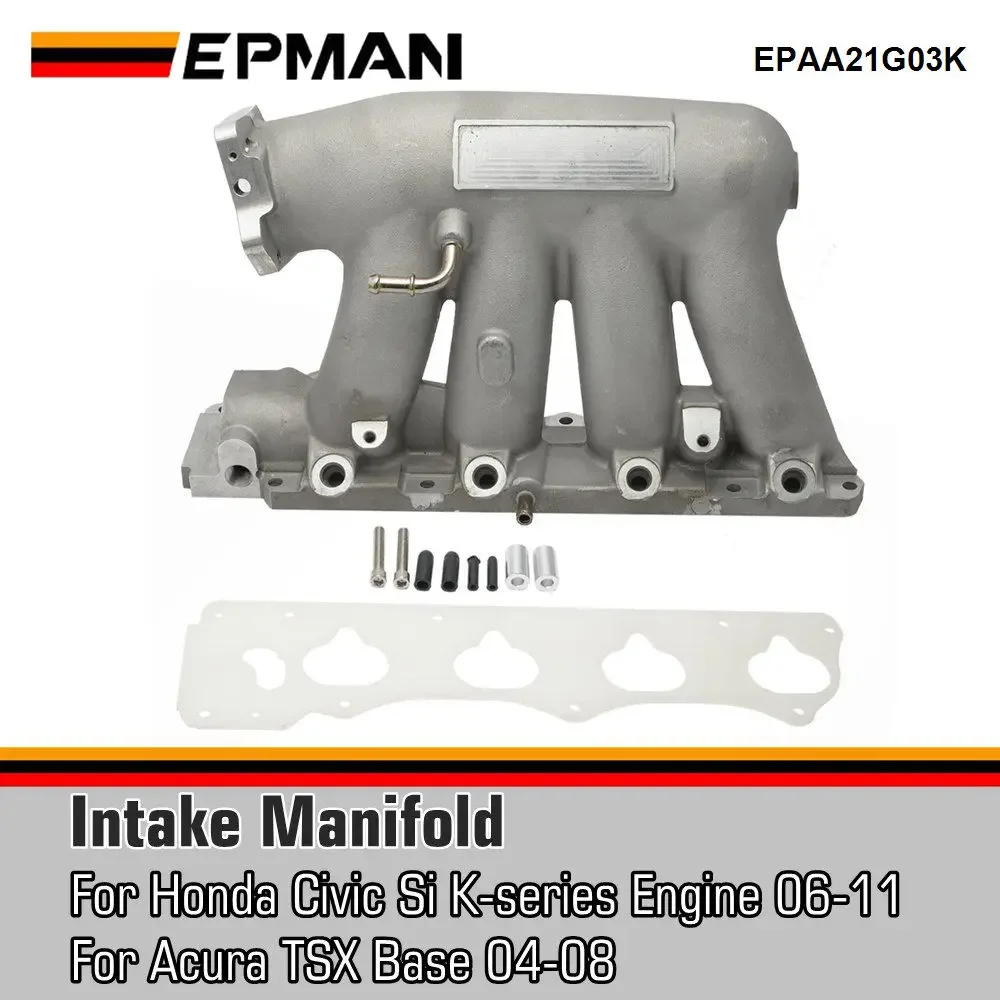The image showcases a gray intake manifold designed for the Honda Civic Si K series engine (2006-2011) and the Acura TSX base model (2004-2008), with the part number EPAA21G03K clearly visible at the top right. The manifold has a distinctive design, resembling an elephant with four cylindrical legs, each featuring screw holes at their base. Above the manifold, the brand name "EPMAN" is displayed alongside three colored stripes - yellow, black, and red. The same three-colored stripe pattern is repeated below the manifold, followed by the bold text "Intake Manifold" over a light gray backdrop. The entire image is set against a clean, white background.